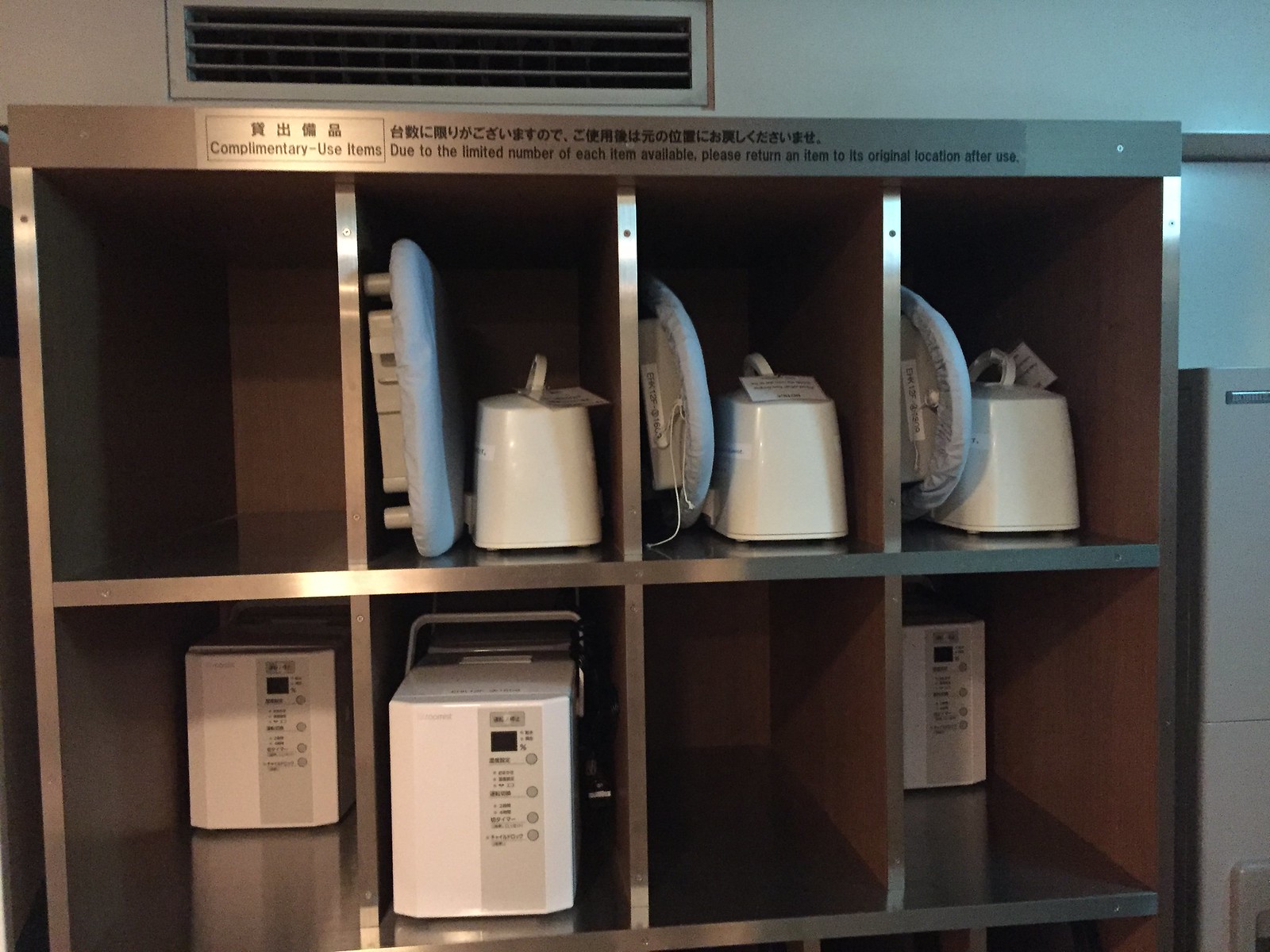The photograph showcases a shiny, silver-colored storage unit featuring eight compartments arranged in a four-by-two grid. Each of the compartments, labeled as complimentary use items, contains various devices available for shared use. Text in English at the top instructs users to return items to their original locations due to their limited availability. These instructions are also written in a foreign language, either Japanese or Chinese, above the English text. The background is a gray wall with a rectangular vent positioned above the storage unit.

The three compartments on the top row contain devices that resemble a tiny fold-up portable ironing board with a light blue cover, standing upright. The bottom row features similar white plastic boxes with buttons, possibly housing items such as irons. Six compartments have appliances, while two compartments remain empty. Despite the detailed descriptions, the exact purpose of each device remains unclear.